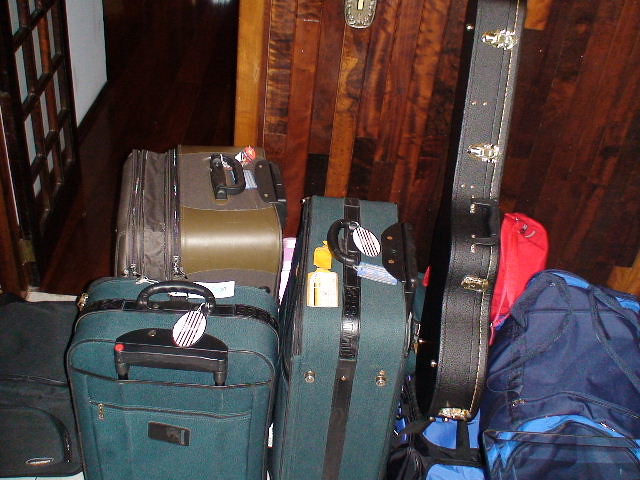The image depicts a collection of various luggage pieces, seemingly gathered for travel either from an arrival or prior to a departure. The luggage is arranged neatly against a wooden wall with vertical panels, and the scene includes an open wooden door with glass panels on the upper left, leading to a room with a dark hardwood floor and white walls.

Centrally, there are four suitcases: two tall, teal green rolling suitcases, a tall brown rolling suitcase, and a smaller carry-on style green suitcase. Also included is a black guitar case standing prominently, leaning on the wall, partially resting on a light blue bag. To the right of the guitar case, there is a blue duffel bag, and behind it, a red backpack can be seen. On the far left, a black bag is positioned closest to the wall. The floor in this setting is wooden, adding a warm, cohesive element to the arrangement.